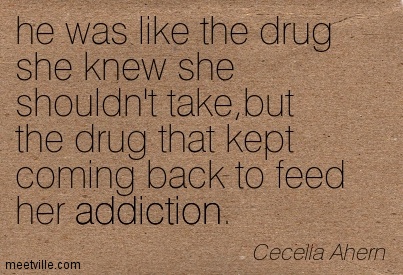The image features a quote in all lowercase, black text on a textured brown background that resembles cardboard. The text reads:

"he was like the drug.
she knew she
shouldn't take, but
the drug that kept
coming back to feed
her addiction."

This quote is left-centered on the background. In the lower left-hand corner, there's a website address: meetville.com. In the lower right-hand corner, in italics, it is attributed to Cecilia Ahern. The entire quote appears against the grainy, cardboard-like background without any additional colors or imagery. The image has a landscape orientation.